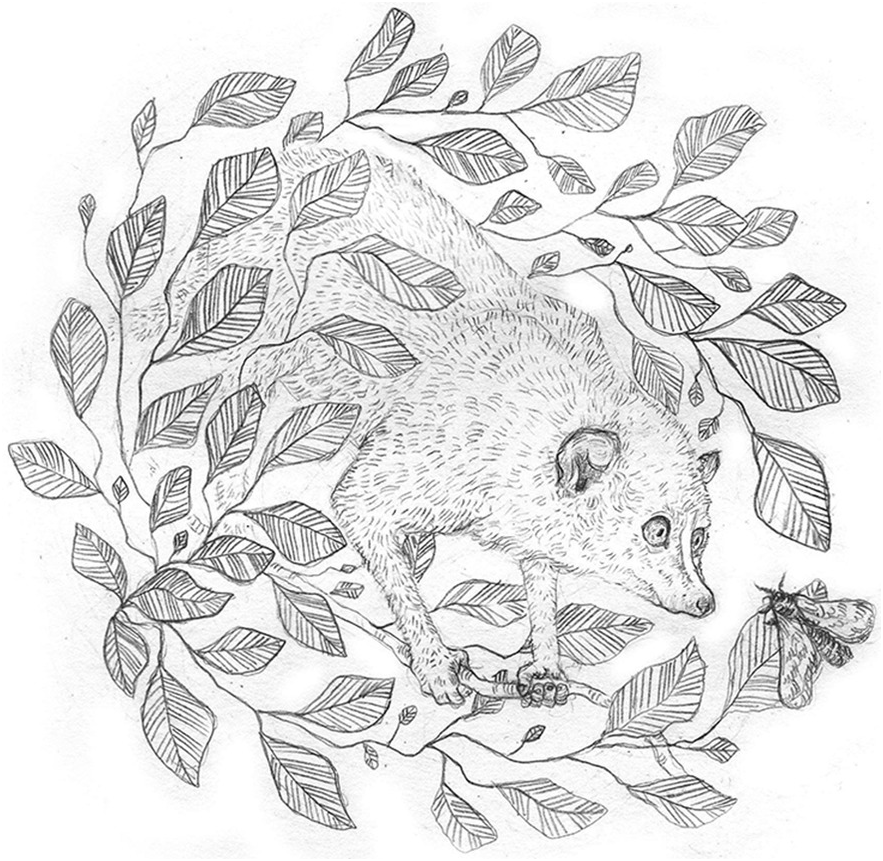This hand-drawn, black and white artwork depicts a circular arrangement of soft, light gray leaves, meticulously crafted to form a frame around the central subject. At the heart of the composition, a delicate, furry creature resembling either a small rodent or a sugar glider clings to a slender branch. Its large, expressive eyes are intently fixed on a butterfly perched on one of the outer leaves. The creature, which exudes an innocent and harmless demeanor, is covered in fine, light gray hairs and features a small snout with prominent ears. Despite the lack of vivid stripes, the intricate pencil strokes used in the drawing highlight the artist’s dedication to detail. The scene conveys a sense of quiet focus as the gentle creature, about 10 inches in length, contemplates the small winged insect within the leafy enclosure.